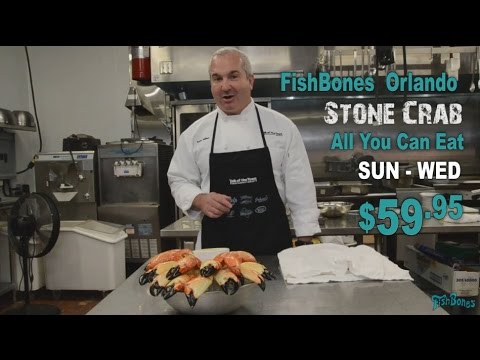The image is a detailed scene from a television or online advertisement for Fish Bones Orlando, emphasizing their Stone Crab all-you-can-eat offer available from Sunday to Wednesday for $59.95. Central to the image is a bald, elderly Caucasian chef, dressed in a classic white chef coat and blue apron. He stands prominently in a commercial kitchen filled with various shiny, silver-stainless-steel machinery, including an area for soft-serve ice cream and cooking equipment like grills and ovens. In front of him, slightly off-center, is a bowl filled with numerous crab legs resting on a table. The text on the right side of the image features green and white fonts, alternating to convey the key promotional details: "Fish Bones Orlando," "Stone Crab," "All You Can Eat," "Sun-Wed," and "$59.95." The entire scene is framed with black widescreen bars at the top and bottom, enhancing its cinematic style. The background features more kitchen apparatus and utensils, adding to the busy, authentic restaurant atmosphere. The color palette includes black, white, gray, brown, pink, orange, yellow, light blue, and red, conveying a lively and appealing visual presentation.